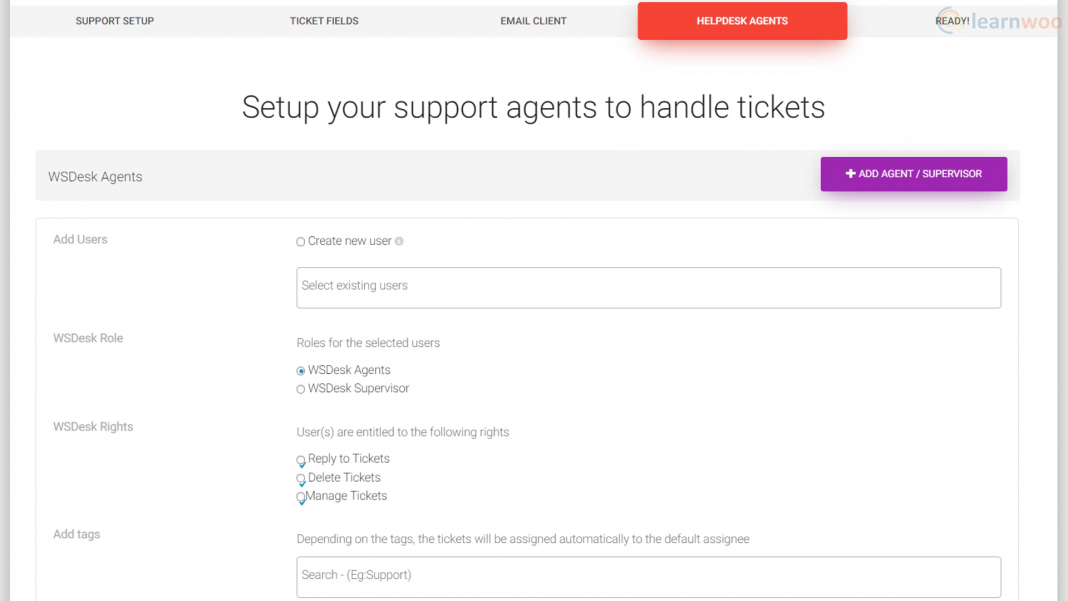The image comprises multiple sections, each with distinct elements and labels, organized in a structured layout to provide detailed instructions and functionalities for setting up support agents in a help desk system.

At the top of the image, there's a horizontal gray border spanning across the width. Below this border, there is a support setup section labeled "Ticket Fields" followed by "E-mail Client." 

Beneath these labels, there is a prominent red box with white text reading "Help Desk Agents." Below this, the text transitions to several colors on a white background: "Ready" in black, "Learn" in blue, "Who" in red. Following this, in black text on the white background, it states, "Set up your support agents to handle tickets."

The middle section contains a gray box with dark gray text labeled "WS Desk Agents." Adjacent to this is a purple rectangular button with white text that reads "Plus, Add Agent/Supervisor."

In the lower part of the image, there is another gray box with an incomplete gray outline, also on a white background. This section appears to be divided into different parts. It lists several options:
- Add Users
- WS Desk Row
- WS Desk Rights
- Add Tags

Following these options is a segment labeled "Create New Users." Here, user roles can be selected, illustrated by two circles with white interiors and gray outlines, labeled "WS Desk Agents" and "WS Desk Supervisor." When a circle is selected, its interior turns blue, indicating that the user is entitled to specific rights including applying to tickets, deleting tickets, and managing tickets.

Lastly, there is a note mentioning that tickets will be automatically assigned to the default assignee based on the tags applied.

The detailed setup instructions and various sections are laid out to facilitate the configuration of support agents effectively, ensuring they have the necessary permissions to manage tickets within the help desk system.